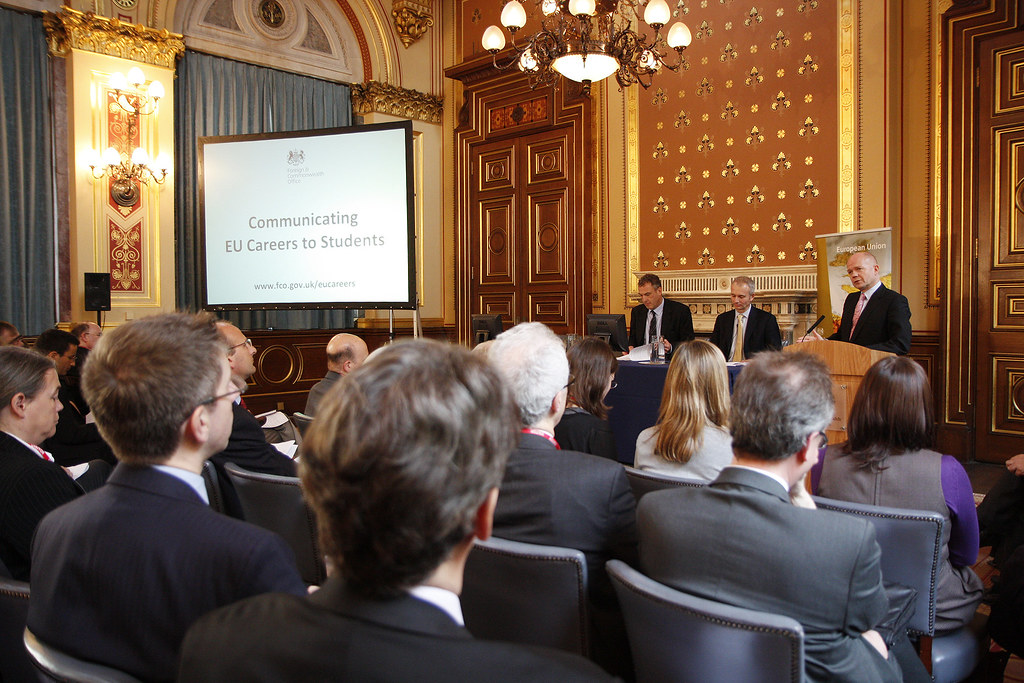The image depicts an ornate conference room filled with a professionally dressed audience, predominantly in black suits, seated in rows of blue leather chairs. Toward the front of the room, to the center left, a large white projection screen with a black border displays the text "Communicating EU Careers to Students," along with a website, www.fco.gov.uk, though some finer details are blurry. The screen also features a small, faded emblem at the top. The backdrop includes a brown wall adorned with blue curtains and elaborate yellow lighting fixtures. A chandelier with numerous lights hangs prominently from the ceiling. In the foreground, three men in suits are positioned; two are seated at a table draped with a dark tablecloth, while the third stands behind a light wooden podium equipped with a microphone. The room also features two large ornate doors on the left and right sides of the background. This appears to be a formal event, likely a political or local government meeting.